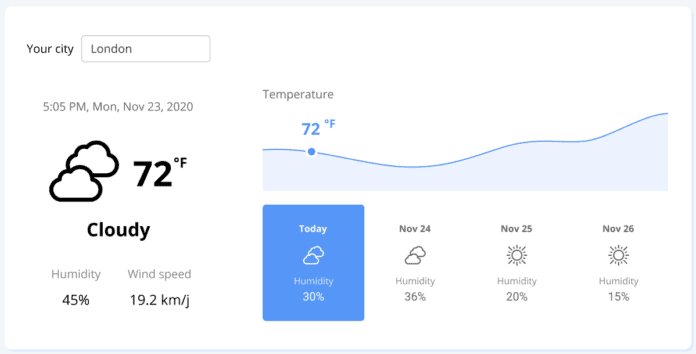Photograph of the London skyline taken at 5:05 p.m. on Monday, November 23rd, 2020. The temperature at that moment was 72°F with a partially cloudy sky. The humidity was recorded at 45%, and the wind speed was 19.2 kilometers per hour. The weather forecast for the following days is as follows: 

- November 24th: Partly cloudy with a humidity of 36%
- November 25th: Sunny with a humidity of 20%
- November 26th: Sunny with a humidity of 15%

The cityscape is beautifully illuminated under the soft, late afternoon light, with the iconic architecture of London silhouetted against the sky.